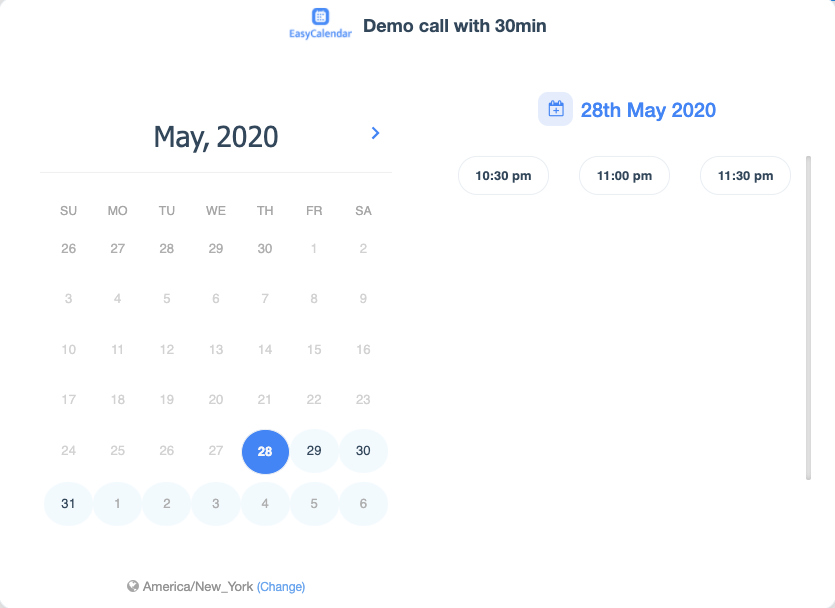This image is a detailed screenshot of a calendar website interface. The main focus of the screen is on the left side, displaying the entire month of May 2020 in a grid format against a white background. The top of the calendar is labeled "May 2020". Days of the week are abbreviated to the first two letters—Su, Mo, Tu, We, Th, Fr, Sa—and listed horizontally.

The calendar grid begins on April 26 and extends to June 6, indicating adjacent months. Days from April 26 to April 30, and June 1 to June 6, are in gray text. Key dates within May are highlighted differently: May 28 is marked with a blue circle and white text, while May 29 to May 31 are shown with gray circles and black text, and May 1 to May 6 are displayed with gray circles and gray text.

To the right of the calendar, there is a sidebar featuring detailed event options. The date "28th May, 2020" is highlighted in blue text, accompanied by a small blue calendar icon with a white plus sign. Below this, three selectable time options—10:30 PM, 11:00 PM, and 11:30 PM in black text—are displayed within oval-shaped buttons. 

At the top center of the image, the website logo "Easy Calendar" is presented in blue text, above which a small blue icon with a white calendar can be seen. Additionally, the text "Demo Call with 30 men" appears in black just below the logo. There is a scroll bar located on the right side of the interface, providing further navigation options.